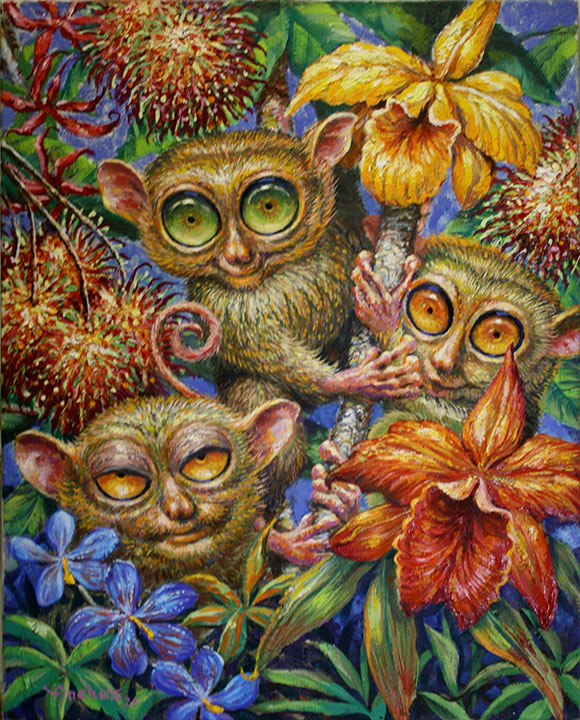In this vibrant and detailed oil painting by Richard Anchetta, three expressive tarsiers are depicted having a playful time among a lush and colorful background. The composition features a tall tree stem crowned with a big yellow flower, which all three tarsiers are gripping onto, set against a vivid tapestry of various flowers and foliage. The top-middle tarsier has striking big green eyes and wears a broad smile, exuding playful energy. To the right, another tarsier with orange and yellow eyes appears to be whistling, its lips puckered in a suggestive manner. Below them, a sleepy-eyed tarsier with its eyelids halfway shut and matching orange and yellow eyes looks content and serene. The background is brimming with an array of colors including blue, red, orange, yellow, and green. Notably, there are pretty blue flowers near the bottom left, a giant red-orange-yellow flower in front of the right tarsier, and clusters of bushy, round, plant-like shapes interspersed with green ferns throughout. The painting's psychedelic color scheme and the tarsiers' bug-eyed expressions contribute to a drug-inspired, hippie art aesthetic, capturing a surreal and whimsical scene in portrait orientation.